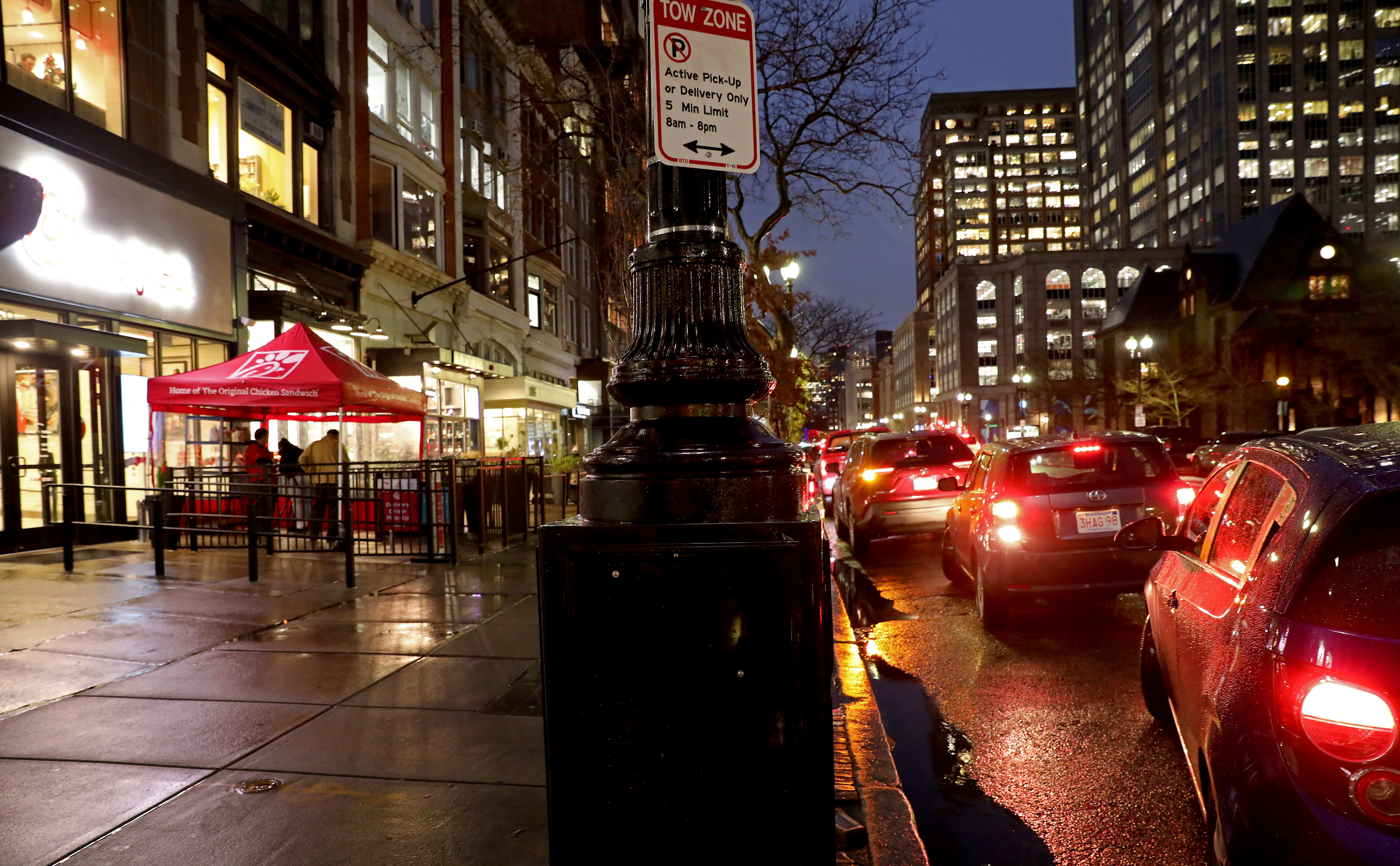A bustling urban scene is captured in this photograph. Dominating the center bottom is a large, black, square base of a pole, from which a pole rises vertically. Affixed to the pole is a tow-away sign, white with a prominent red stripe at the top, clearly warning about parking restrictions. To the left, a gray concrete sidewalk, composed of large, square sections, is visibly wet, likely from a recent rain. Further left, tall city buildings add to the urban skyline. On the right side of the image, a street lined with cars, all at a standstill, their taillights glowing a vivid red, suggesting heavy traffic. The upper right-hand corner reveals a couple of office buildings, their windows aglow with interior lights. A striking feature in the center of the background is a tree, leafless with its intricate branches silhouetted against a twilight sky painted in rich purples. The entire scene is enveloped in a moody, atmospheric ambiance that highlights the interplay between urban infrastructure and the early evening light.